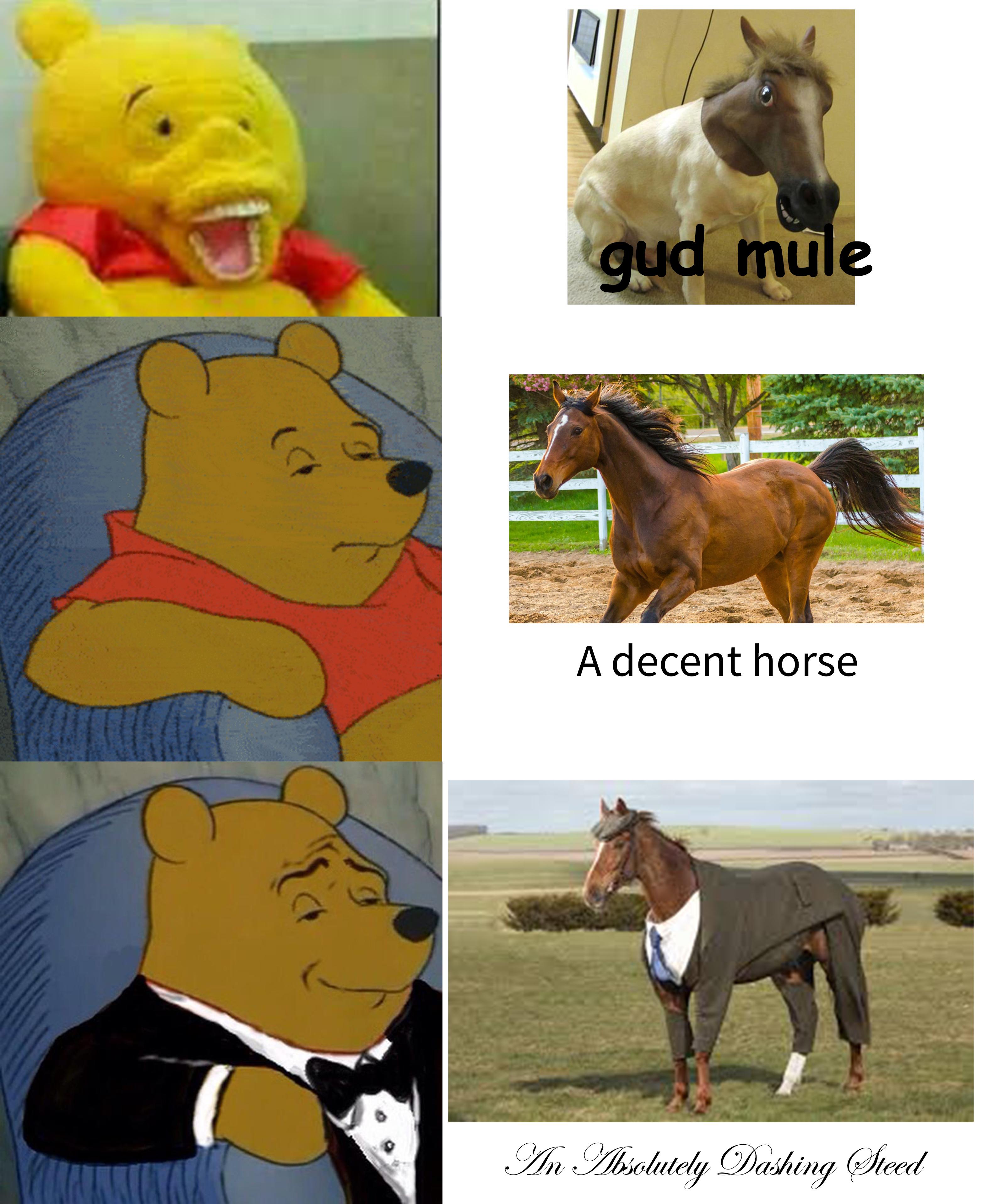The image features a humorous comparison between cartoon bears and real-life horses. At the top left, there is a yellow stuffed bear with a red shirt and an open-mouthed grin, showing a full set of teeth. It is paired on the right with a cartoon mule labeled "Gud Mule," which is depicted with brown and white coloring. In the middle left, another cartoon bear, dressed in a red shirt, looks tired while sitting in a chair. Its counterpart on the right is a brown horse, described as "Decent Horse," which is shown galloping past a white fence. At the bottom left, a bear in a black tuxedo with a white shirt and black bow tie sits in a blue chair. To the right of this bear is a brown horse dressed in a stylish gray suit and hat, and the caption beneath reads "Absolutely Dashing Steed." The background exhibits colors like green, brown, white, blue, and red.